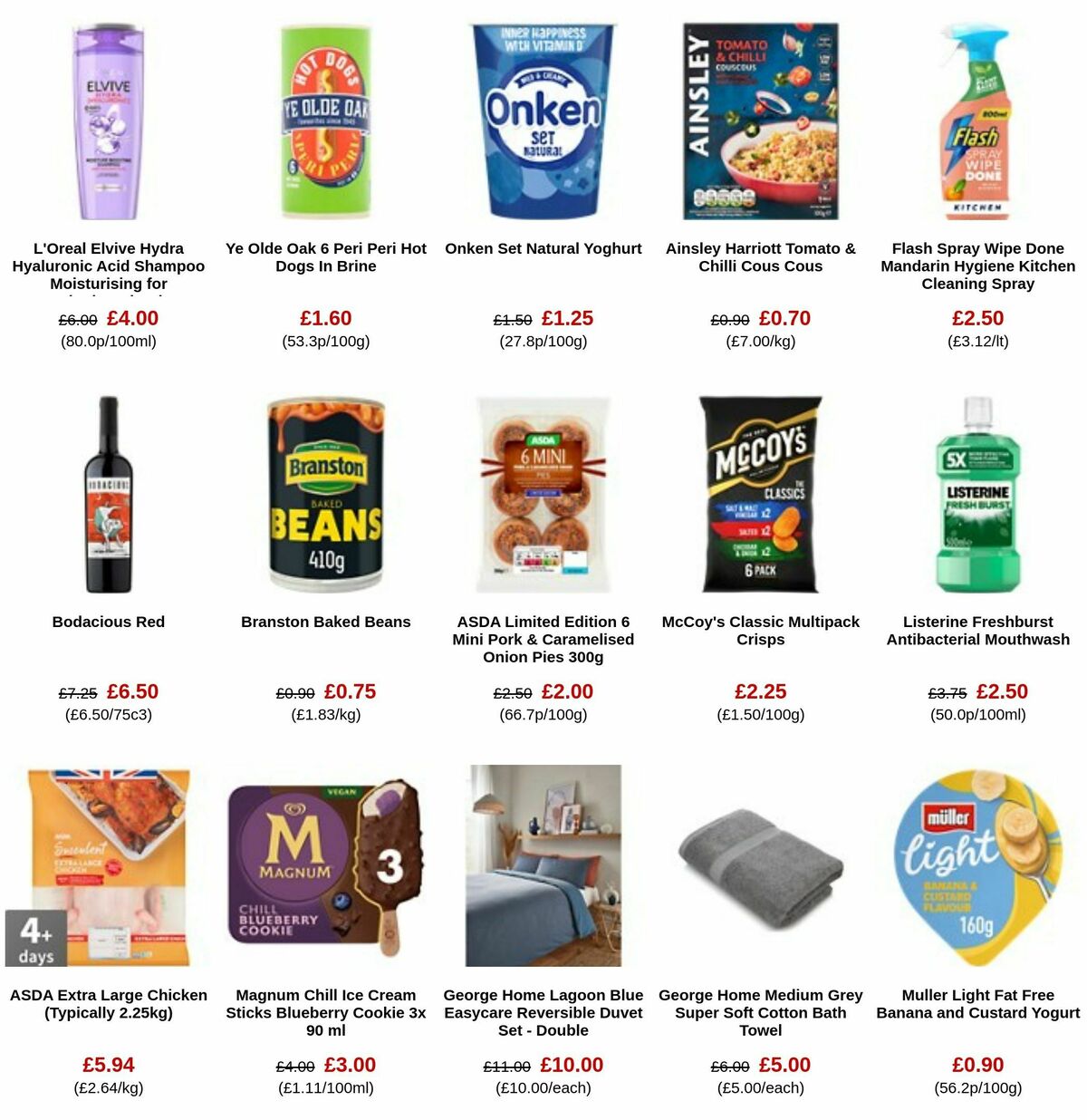**Detailed Caption:**

This screenshot captures a web page showcasing a diverse range of products, several of which have prices that have been marked down indicating discounts. 

- **Top Row:**
  1. **L'Oreal L'Viv Hydra Hyaluronic Acid Shampoo Moisturizing**
  2. **Yale Oak and Peri Peri Hot Dogs in Brine**
  3. **On Conset Natural Yogurt**
  4. **Ainsley Harriet Tomato and Chili Couscous**
  5. **Flash Spray Wipe Done Mandarin Hygiene Kitchen Cleaning Spray**

- **Second Row (Middle Row):**
  1. **Bodacious Red Wine**
  2. **Branston Beans**
  3. **ASDA Limited Edition Mini Pork Caramelized Onion Pies**
  4. **McCoy's Classic Multipack Crisps**
  5. **Listerine Fresh Burst Antibacterial Mouthwash**

- **Bottom Row:**
  1. **ASDA Extra Large Chicken**
  2. **Magnum Chill Ice Cream**
  3. **George Home Lagoon Blue Easy Care Reversible Duvet**
  4. **George Home Medium Gray Super Soft Cotton Bath Towel**
  5. **Mueller Light Fat-Free Banana and Custard Yogurt**

This organized display provides a clear view of various products ranging from personal care items and food products to household essentials, each carefully arranged for easy browsing.